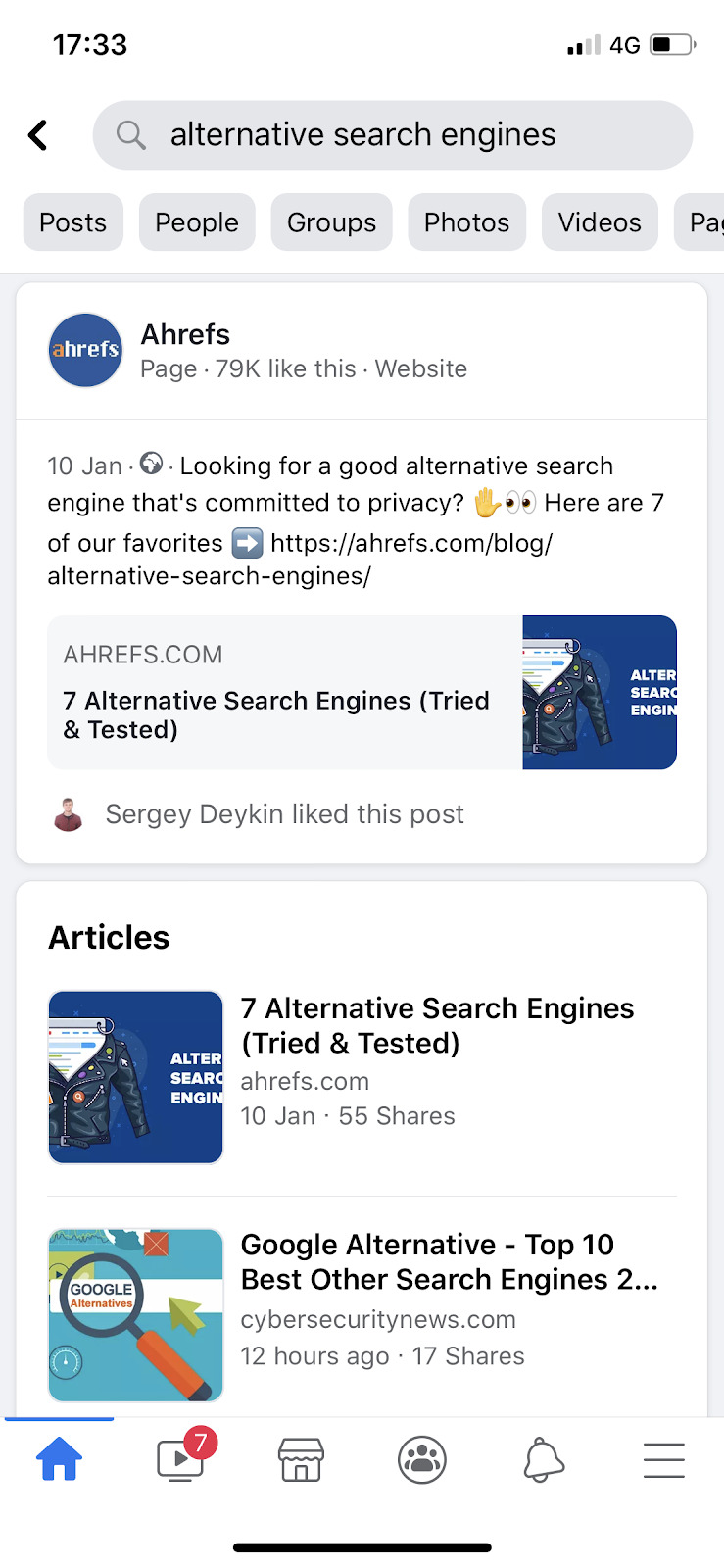A screen capture from an app displayed on a standard iPhone screen. At the top, there is a ribbon showing the time on the left and indicators for battery life, signal bars, and other standard icons on the right. Below this, the central part of the app displays a search that has been performed.

The search bar contains the phrase "Alternative search engines." Beneath the search bar, there are several navigation buttons labeled "Posts," "People," "Groups," "Photos," and "Videos."

The first visible search result is from "AHREF.com," boasting that 79,000 users like the website. The snippet reads, "Looking for a good alternative search engine that is committed to privacy? Here are seven of our favorites," followed by a link to the article titled "Seven Alternative Search Engines Tried and Tested."

Following this, there is another section labeled "Articles." The first article is a repeat of the previously mentioned one from AHREFS.com, posted on January 10 with 55 shares. Below that, another article titled "Google Alternative: Top 10 Best Search Engines" from cybersecuritynews.com is listed, noted to have been posted 12 hours ago with 17 shares. To the left of each article title is a small accompanying icon, likely representing the source or category of the content.